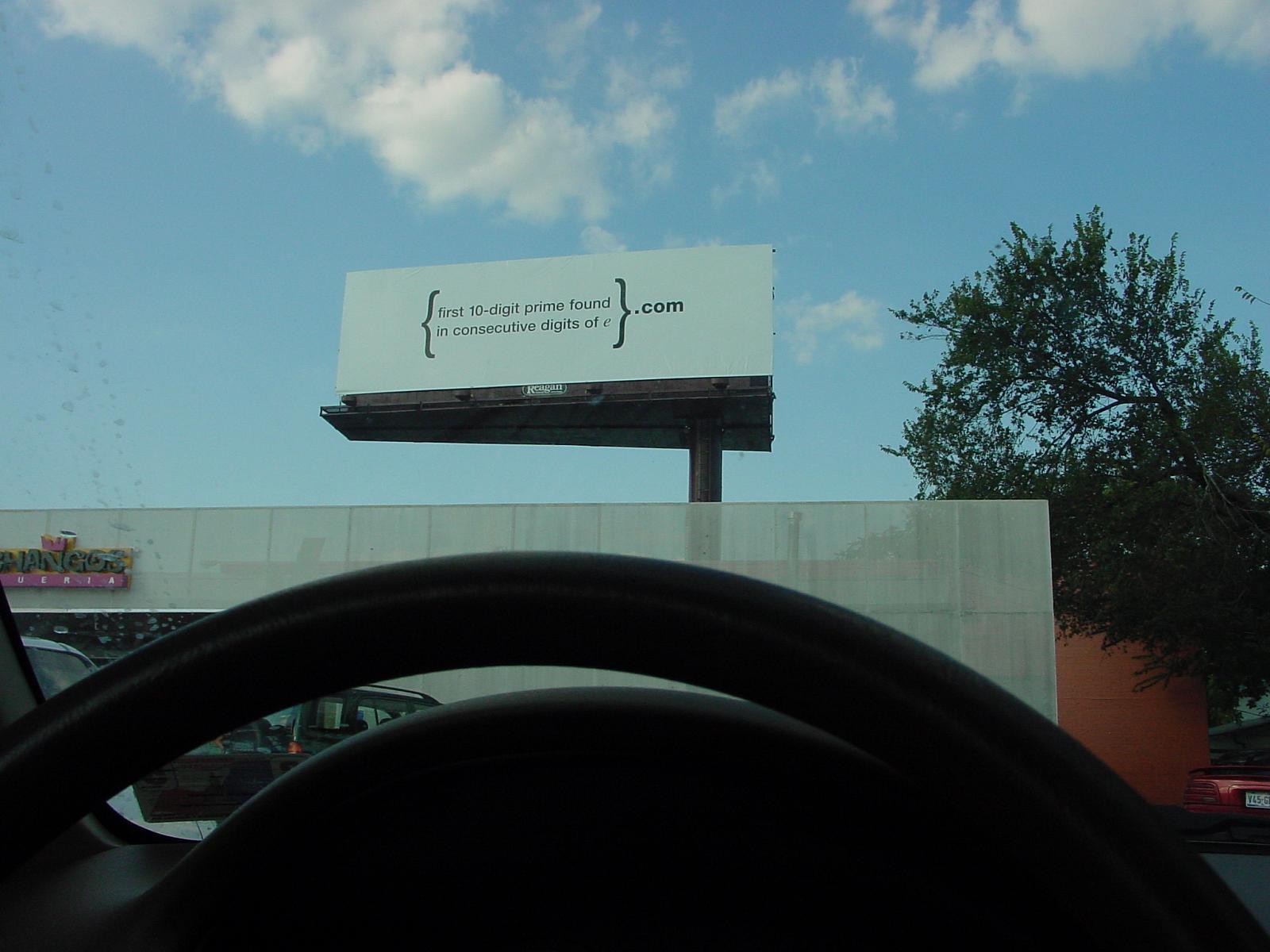A photograph captured from inside a car parked in a lot showcases a multi-faceted scene dominated by a prominent billboard. The billboard, framed with parentheses, boldly reads, "first 10 digit prime found in consecutive digits of e dot com". In the backdrop, beyond the billboard, stands a building with signage indicating it is a Chinese restaurant named 'Shanghai'. The foreground of the image features the interior of the car, including the steering wheel, dashboard, and a glimpse of the windshield's corner, affirming that the scene is viewed from inside the vehicle. Through the windshield, multiple vehicles are visible, including another car and a truck parked alongside. The setting is clearly a parking lot, providing a bustling yet static tableau centered around the enigmatic billboard message.